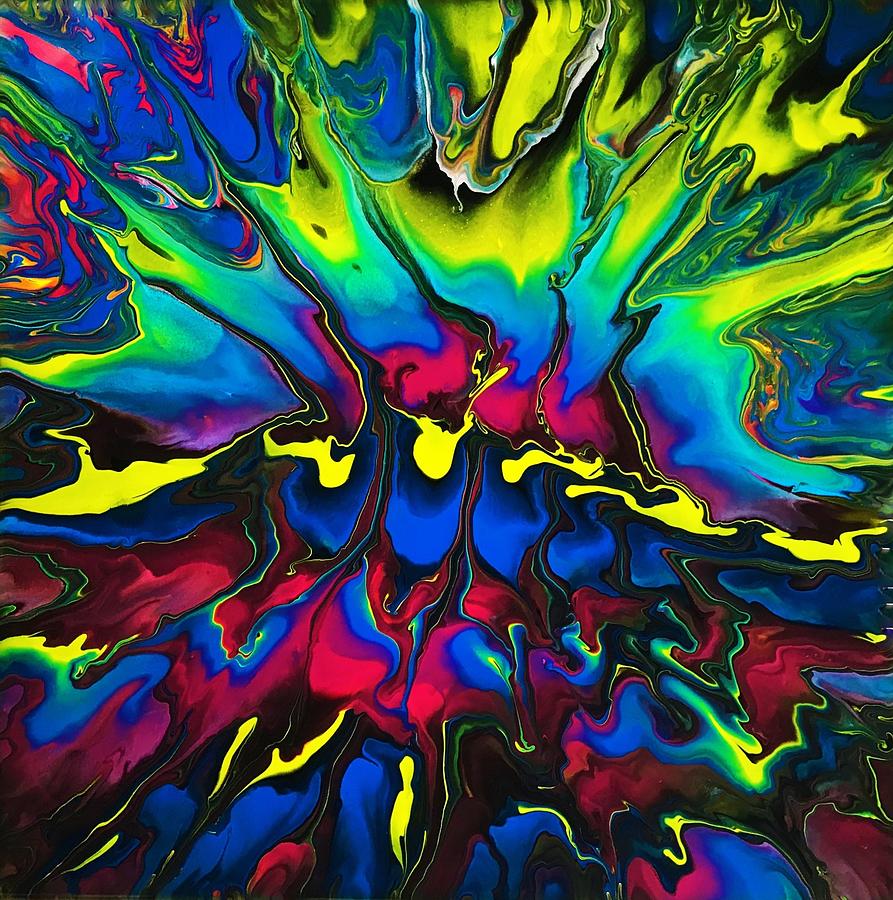This vibrant and energetic abstract painting resembles an acrylic pour with a multitude of bold, primary colors including bright yellow, cobalt blue, and vivid red. Intermingling hues create secondary colors like neon green where blue and yellow overlap, emphasized by dynamic black separations that add depth. The composition seems to radiate from the center in multicolored streaks, puddles, and streaming cells typical of paint pouring, generating a sense of chaotic movement. Additional colors like hot pink, royal blue, fluorescent green, mauve, purple, and dark yellow further enrich the palette. The image is devoid of any text or discernible shapes, focusing purely on the striated, flowing lines and blurred edges that merge toward the periphery, capturing an overall aesthetic of unrestrained, colorful splash art.